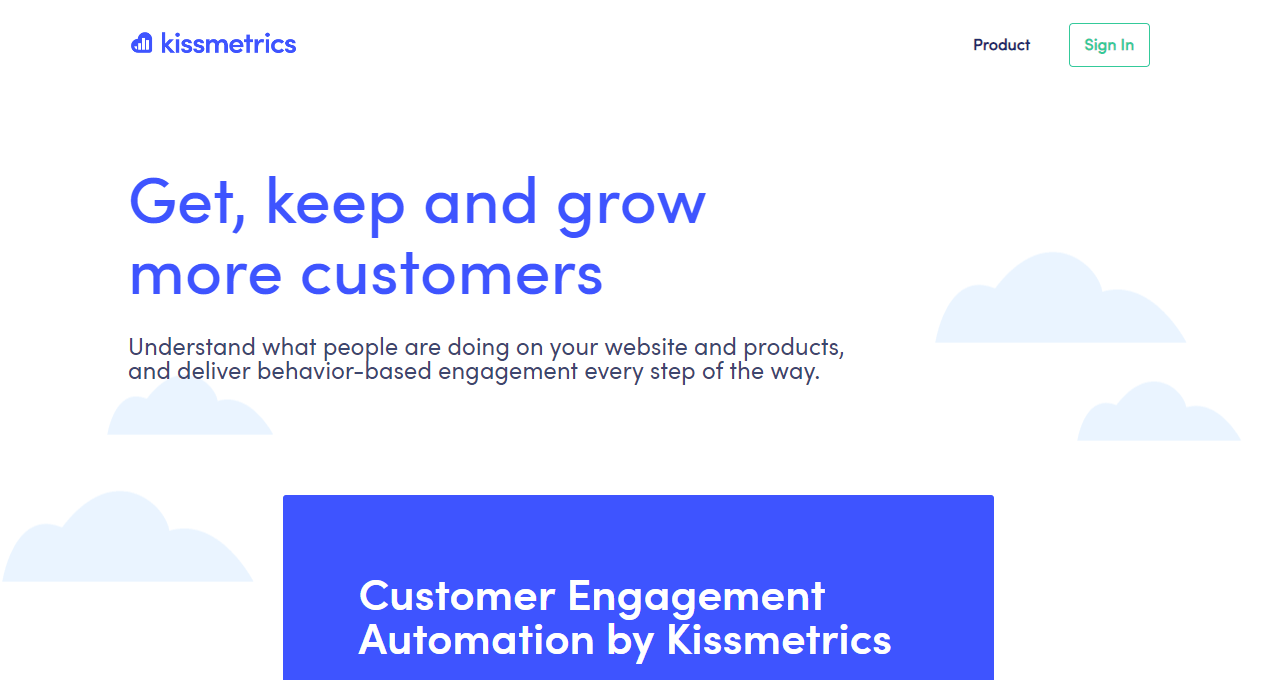The image is a screenshot of a Kissmetrics landing page. In the upper left corner, the Kissmetrics logo is displayed in a light purple color, featuring a side-angled heart with four small bar graphs inside it, followed by the company name in lowercase letters. To the right of the logo, there is a black text button labeled "Product" and a green text button labeled "Sign In," which is enclosed in a thin rectangular box.

The main section of the page prominently displays the text: "Get, keep, and grow more customers," with "more customers" appearing on a second line. Below this, smaller text reads: "Understand what people are doing on your website and products, and deliver behavior-based engagement every step of the way." Underneath this, a purple rectangle contains the text "Customer Engagement Automation by Kissmetrics," although this part appears cut off, suggesting the screenshot is truncated. Overall, the page mostly contains text and lacks a clear call to action, except for the simple "Sign In" button.